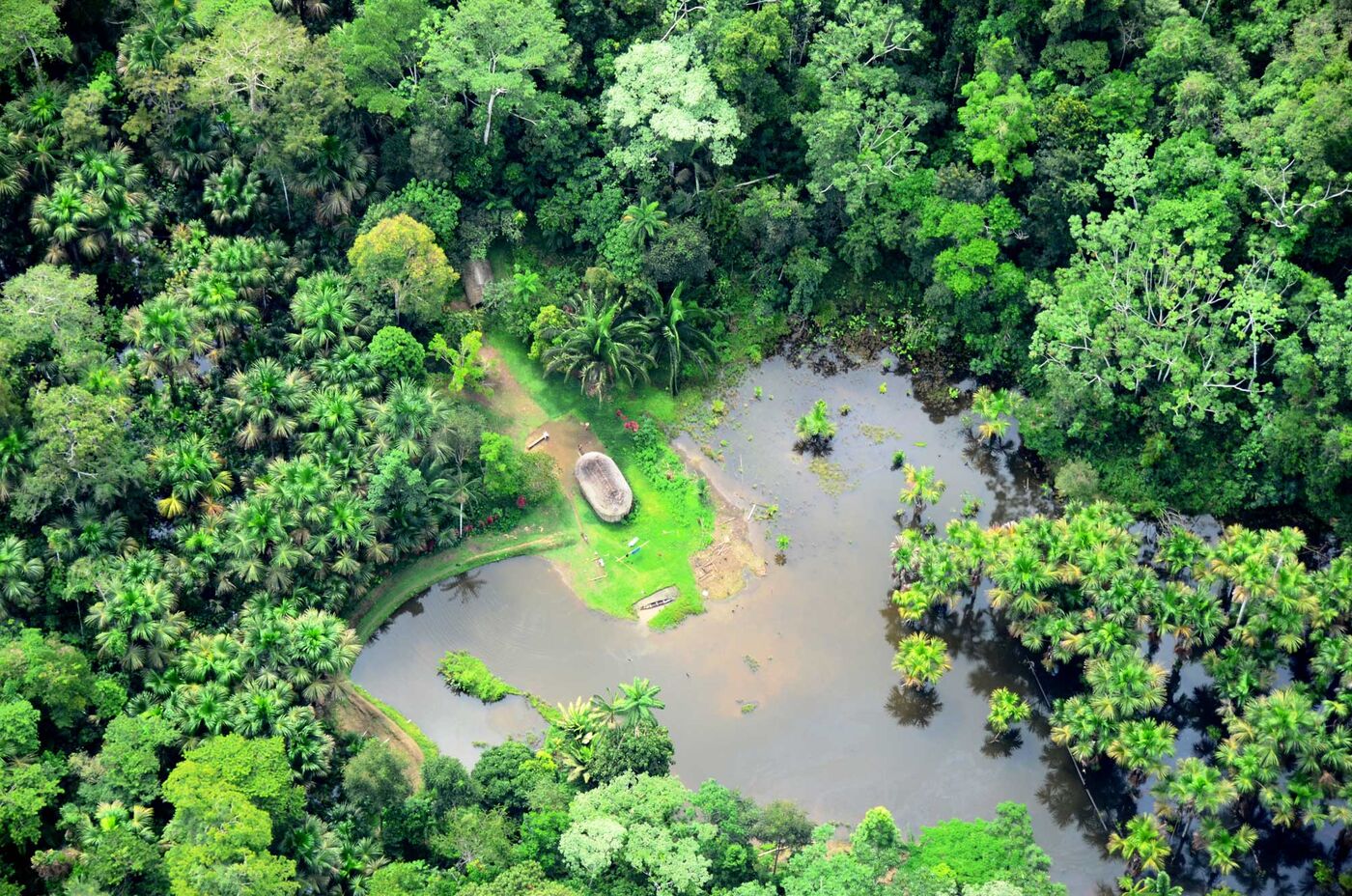This detailed aerial photograph captures a lush, expansive forest with large, distinct trees sprawling out in various directions, indicating they've been there for generations. Dominating the scene is a pond or stream of murky, light brown water, roughly heart-shaped with its top section pointing towards the center bottom of the image. The water appears to have caused some flooding, with the trees along the bottom right partially submerged, suggesting recent heavy rainfall or a storm. Near the top of the heart-shaped body of water, there is a small, cleared area featuring bright green grass, surrounded by a muddy embankment. Centrally situated within this cleared space is a large, oval-shaped rock with an indentation on top, accessible by an adjacent dirt road. The vibrant greenery of the forest, highlighted by numerous palm-like trees, frames this serene yet somewhat swampy landscape, adding layers of rich, natural colors and textures throughout the image.